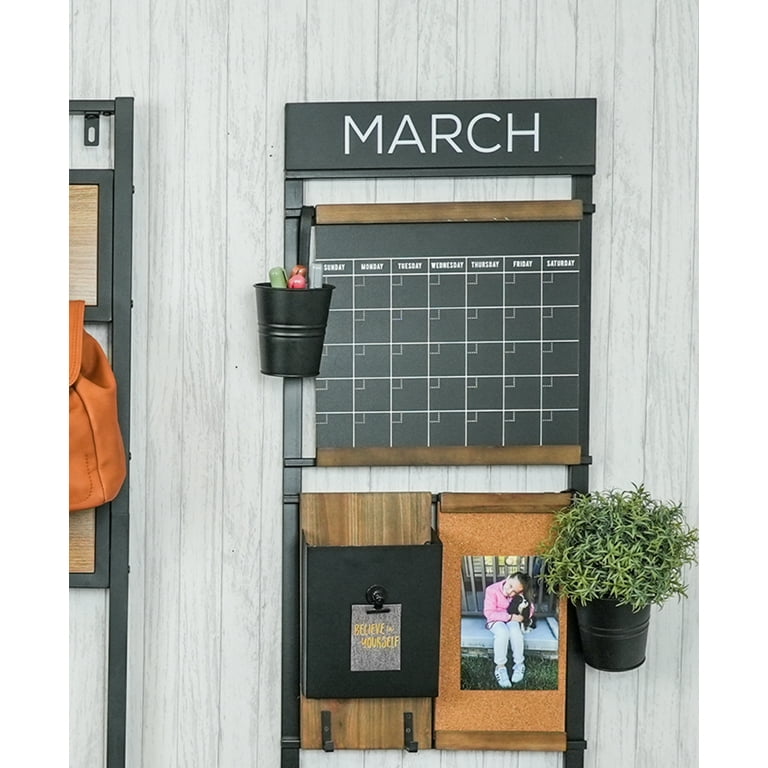The photograph captures a family organizing station mounted on a light gray, white-paneled wall. Dominating the station is a chalkboard calendar with a gray frame. At the top, a removable black rectangular strip with white letters spells out "MARCH." Below this strip, there's a gap revealing the wall before the actual chalkboard section starts. This chalkboard displays a grid, seven boxes wide and five boxes tall, with white writing indicating the days of the week: Sunday, Monday, Tuesday, Wednesday, Thursday, Friday, and Saturday. Each square of the grid contains smaller boxes for individual dates, allowing for flexible monthly arrangement. 

On the left side of the calendar frame, there's a black metal cup holding assorted markers and chalk pens in red, green, and gray. Below the chalkboard section, there's another gap followed by an organizational panel. This panel includes a magnetized clipboard holding a note that reads "Believe in Yourself" and a corkboard featuring a photo of a young girl hugging a puppy. To the left of the clipboard, a black container holds a small green plant, while to the right, there's another black bucket with a spider plant. Adjacent to this organizing station, there appears to be a station for hanging items such as clothes or backpacks, maintaining a consistent style with the primary calendar setup.